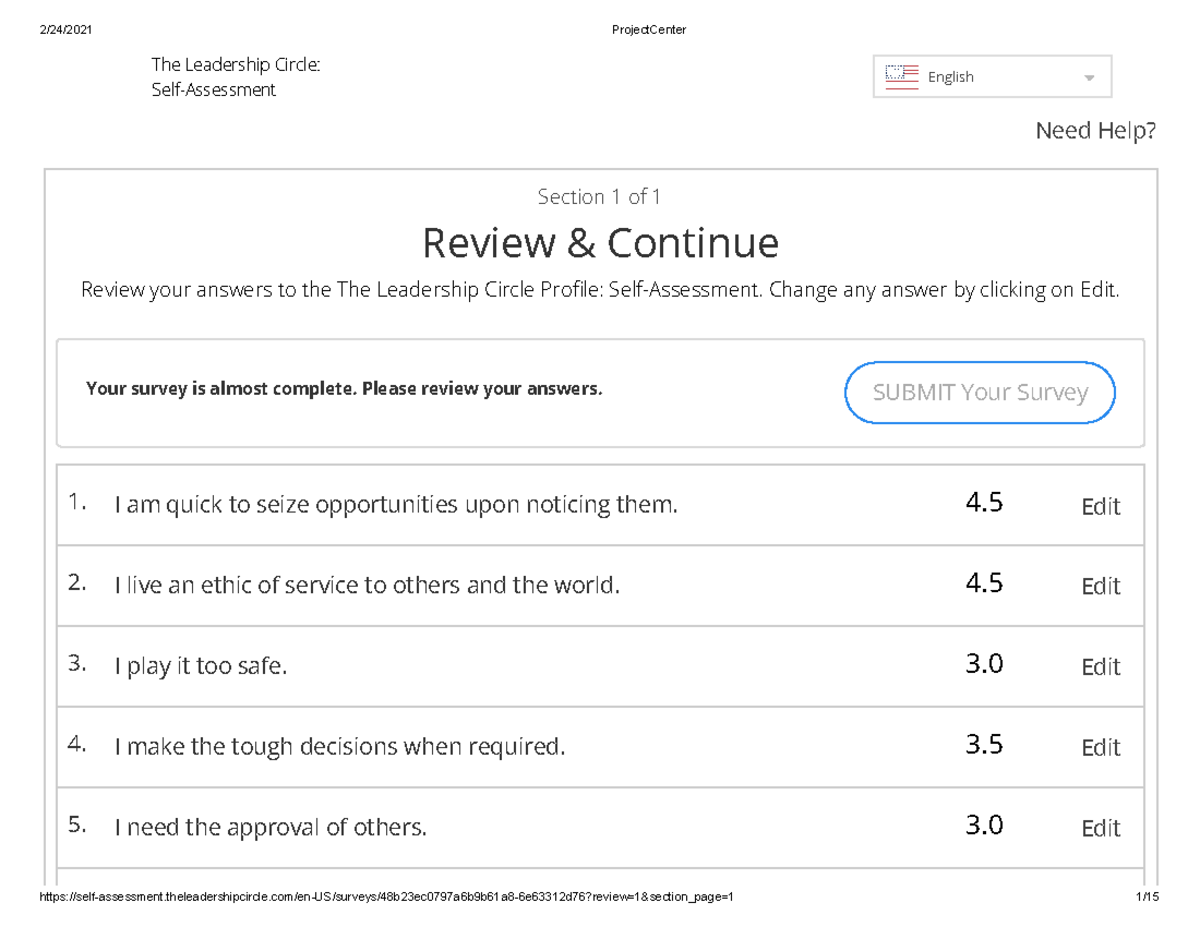The image is a left-to-right horizontal view, seemingly captured from a smartphone or laptop. The background is non-existent, suggesting that the light from the computer screen is in focus. Centrally positioned on the screen is the date "2-24-2021" in black text. Below it, the title "Project Center" is prominently displayed. 

On the left-hand side, there's a section labeled "Leadership Circle Self-Assessment." On the right-hand side, the language option is set to "English," indicated by an American flag icon, with an arrow next to it for changing the language selection. Below this is a black text that reads, "Need help?"

The main content area features a grey box. At the top of the box, the header "Section 101" is highlighted in bold black text, followed by a subheader "Review and Continue" in a slightly less bold black font. The body text instructs to "Review your answers to the Leadership Circle Profile Self-Assessment. Change any answer by clicking on edit." 

Another bold text underneath reads, "Your survey is almost complete. Please review your answers." Adjacent to this is a blue, rounded rectangular button next to a grey side that says, "Submit Your Survey."

The survey features five statements, each with an associated score and edit button:
1. "I am quick to seize opportunities upon noticing them" - scored 4.5.
2. "I live an ethic of service to others in the world" - scored 4.5.
3. "I play it too safe" - scored 3.0.
4. "I make the tough decisions when required" - scored 3.5.
5. "I need the approval of others" - scored 3.0.

Each statement has an edit option for modification.